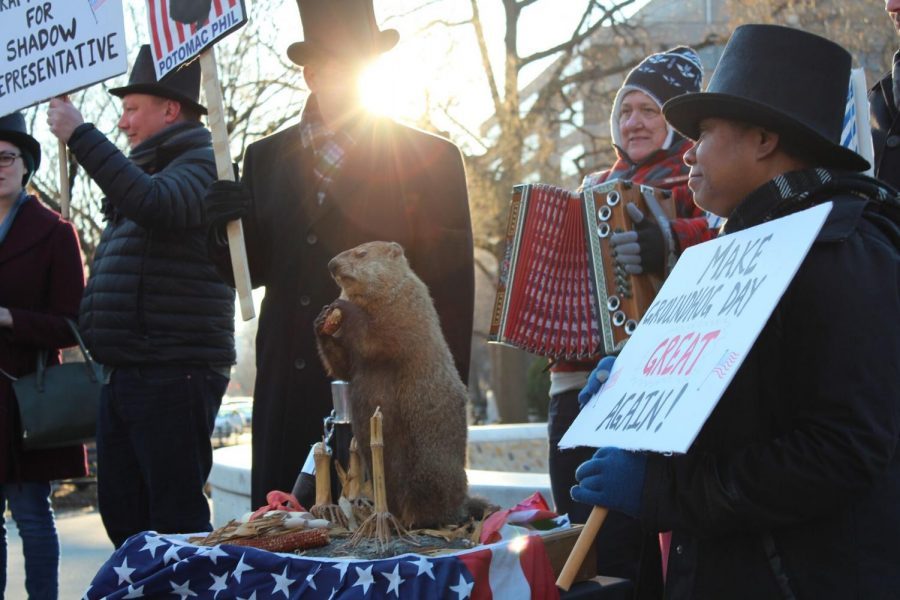In this full-color, horizontally rectangular photograph taken outdoors in the morning during winter, the central focus is a brown groundhog named Potomac Phil, positioned prominently on a table draped with an American flag. Potomac Phil, looking alert and possibly holding a nut, is surrounded by an array of items on the table, including Indian corn and what appears to be bamboo sticks. 

Behind Phil stands a gentleman donning a long black coat, a top hat, and holding a sign that reads "Make Groundhog Day Great Again." A woman to the right, in a red coat and a sock cap, is playing a large red accordion. Around her and scattered throughout the scene are multiple men, each in similar black coats and top hats, one of whom holds a sign partially visible with the words "foreshadow representative." 

The background showcases leafless trees under the bright morning sun, which casts a glow over the man with the "Make Groundhog Day Great Again" sign, slightly obscuring his facial features. The cold weather is evident from the bundled-up individuals, emphasizing the wintry atmosphere of this apparent Groundhog Day celebration.